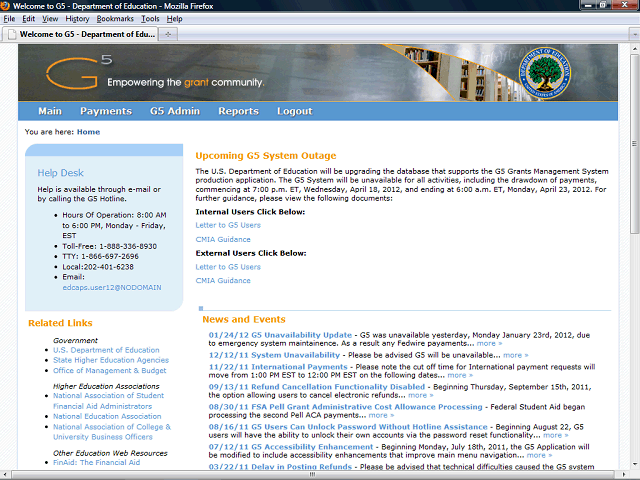The image displays a browser window with the G5 Department of Education interface open in Mozilla Firefox. The interface prominently features the G5 logo, with the tagline "Empowering the Grant Community." At the top of the screen, there's a blue navigation bar with white text, including options for "Main," "Payments," "G5 Admin," "Reports," and "Log Out." Additionally, there's a help desk section offering assistance via email or by calling the G5 hotline. The help desk operates from 8 a.m. to 6 p.m., Monday through Friday, Eastern Standard Time, and provides a toll-free number, TTY number, local number, and email address for support.

A notification is visible about an upcoming G5 system outage. It informs users that the U.S. Department of Education will be performing a database upgrade to support the G5 grant management system's production application. Consequently, the G5 system will be unavailable for all activities, including downloads and payment draws, starting at 7 p.m. Eastern Time on Wednesday, April 18, 2012, and concluding at 6 p.m. Eastern Time on Monday, April 23, 2012. For further guidance, users are directed to click on provided links to view relevant documents. Internal users and external users have separate links for accessing the "Letter to G5 Users" and "CMIA Guidance" documents.